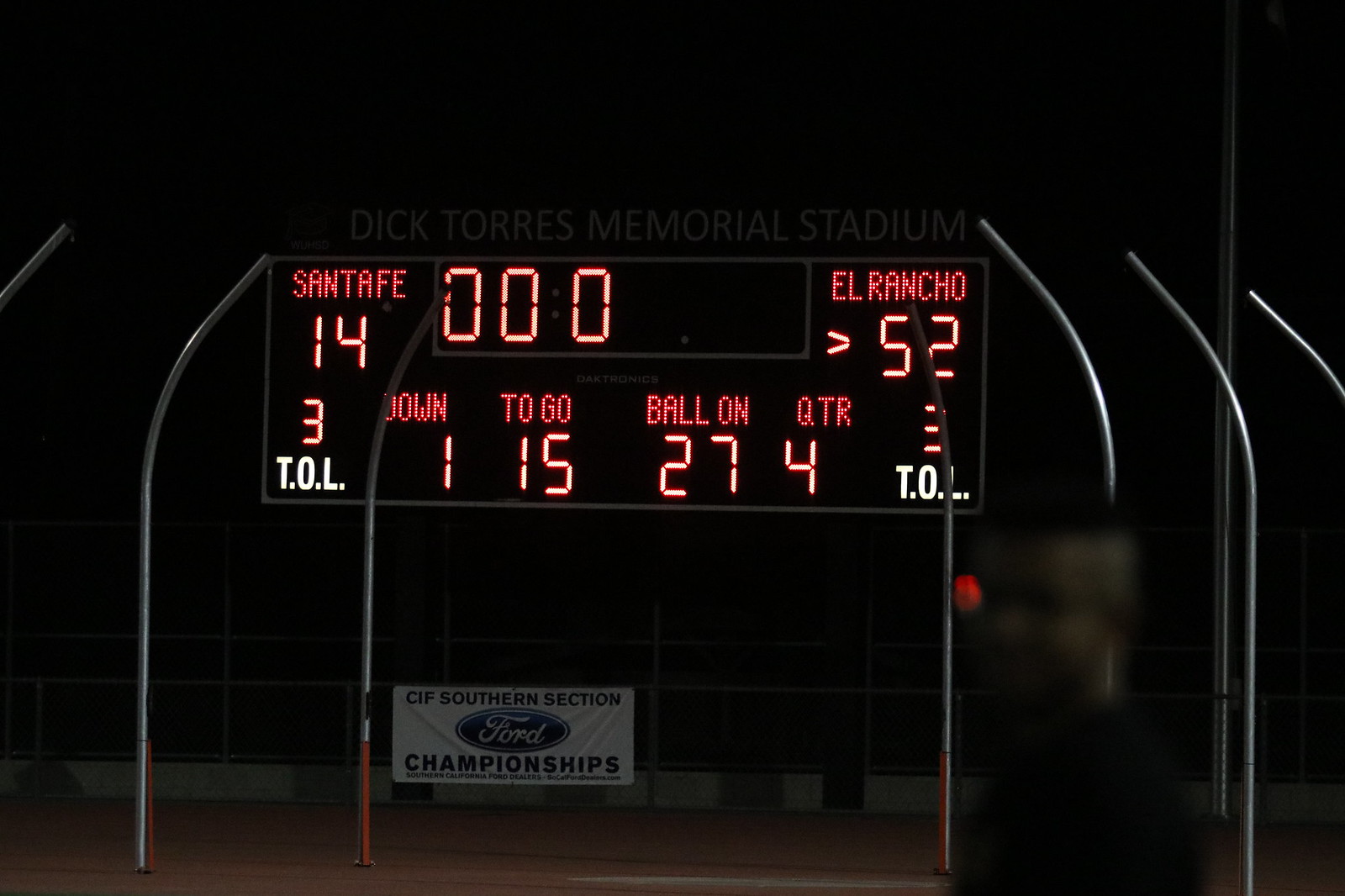This is a well-lit nighttime photograph of a scoreboard at Dick Torres Memorial Stadium, which stands out against a dark background. The scoreboard prominently displays the score of a football game between Santa Fe and El Rancho, with Santa Fe trailing 14 to El Rancho's 52. The game clock reads 0:00, indicating that it is the end of the third quarter, transitioning into the fourth. Additional details on the scoreboard show that it is first down with 15 yards to go, and the ball is on the 27-yard line. Both teams appear to have three timeouts remaining. Below the scoreboard is a fence with a banner that reads "CIF Southern Section Ford Championships," featuring the blue Ford logo. The scene, set in the dark of night, draws attention to the illuminated scoreboard and its detailed information.